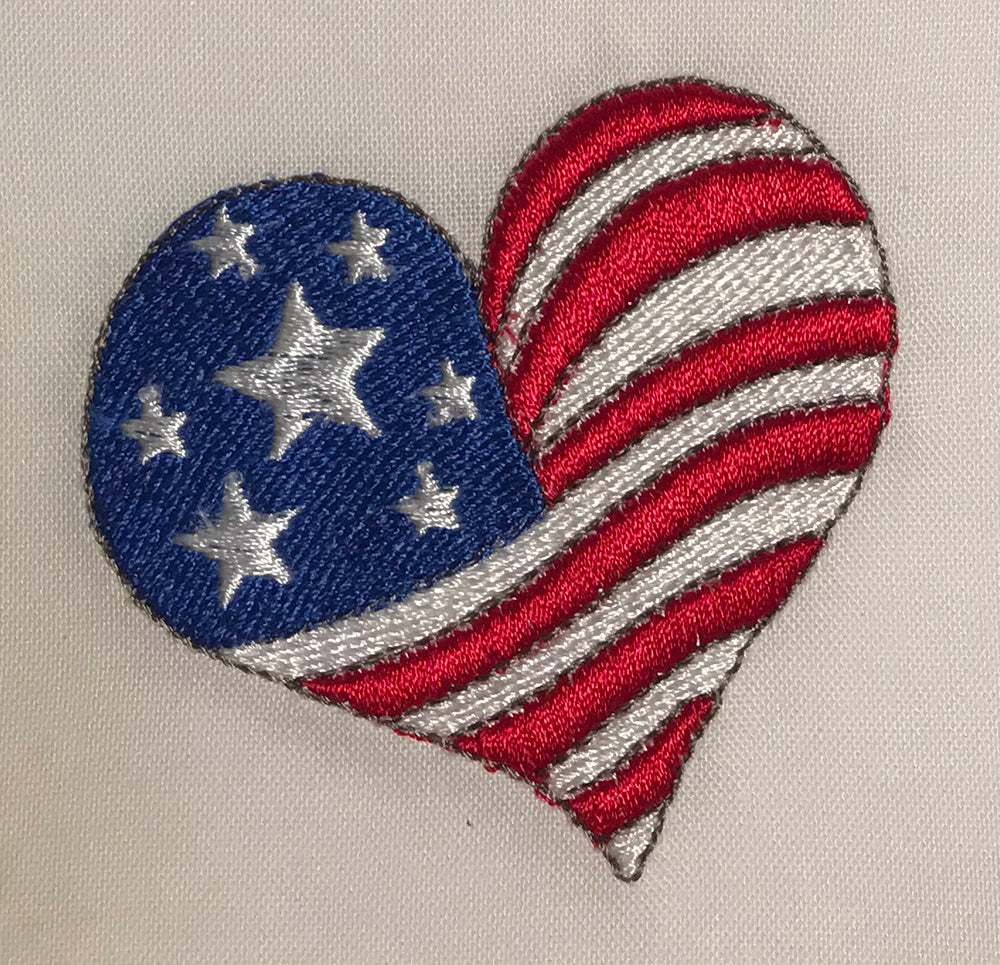This photograph captures an up-close view of a knitted or embroidered American flag in the shape of a heart, positioned slightly diagonally to the left. The heart is intricately woven or quilted into an off-white or light beige fabric. The top left portion of the heart features a blue background with seven stars: one larger silver star in the center and six smaller silver stars surrounding it. The remaining sections of the heart are filled with alternating horizontal red and silver-white stripes, with six red stripes and six white stripes in total. Despite the unconventional shape and slight inaccuracy in the number of stars and stripes, the heart vividly represents the American flag, giving an impression of it waving in the breeze and compressed into a heart form. The detailed stitching and the contrast between the colors highlight the intricate craftsmanship of this embroidered piece.